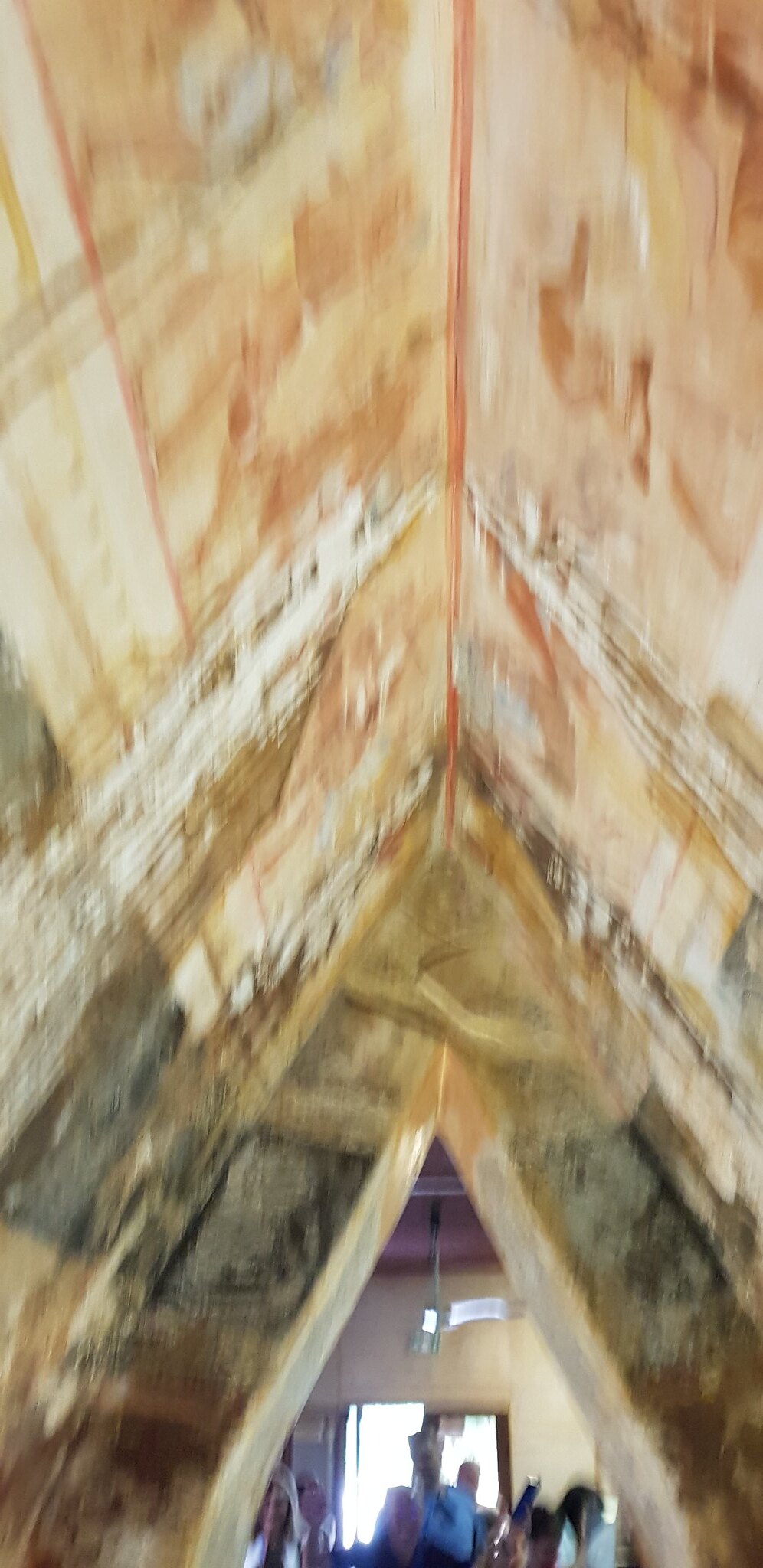The image is extremely blurry, making it difficult to discern specific details. In the background, there is a triangular-shaped area pointing outward, suggesting an indoor setting. A group of people appears in the foreground, though they are also indistinct due to the blurriness. Among them, one person is wearing a white shirt and another a blue shirt, and they seem to be forming a small crowd. Behind them, a door or window is visible, suggesting they are looking towards the camera inside a tent-like structure. The triangular section features a watercolor-textured blend of peach, yellow, orange, green, gray, and brown hues, adding a multi-colored backdrop to the scene.